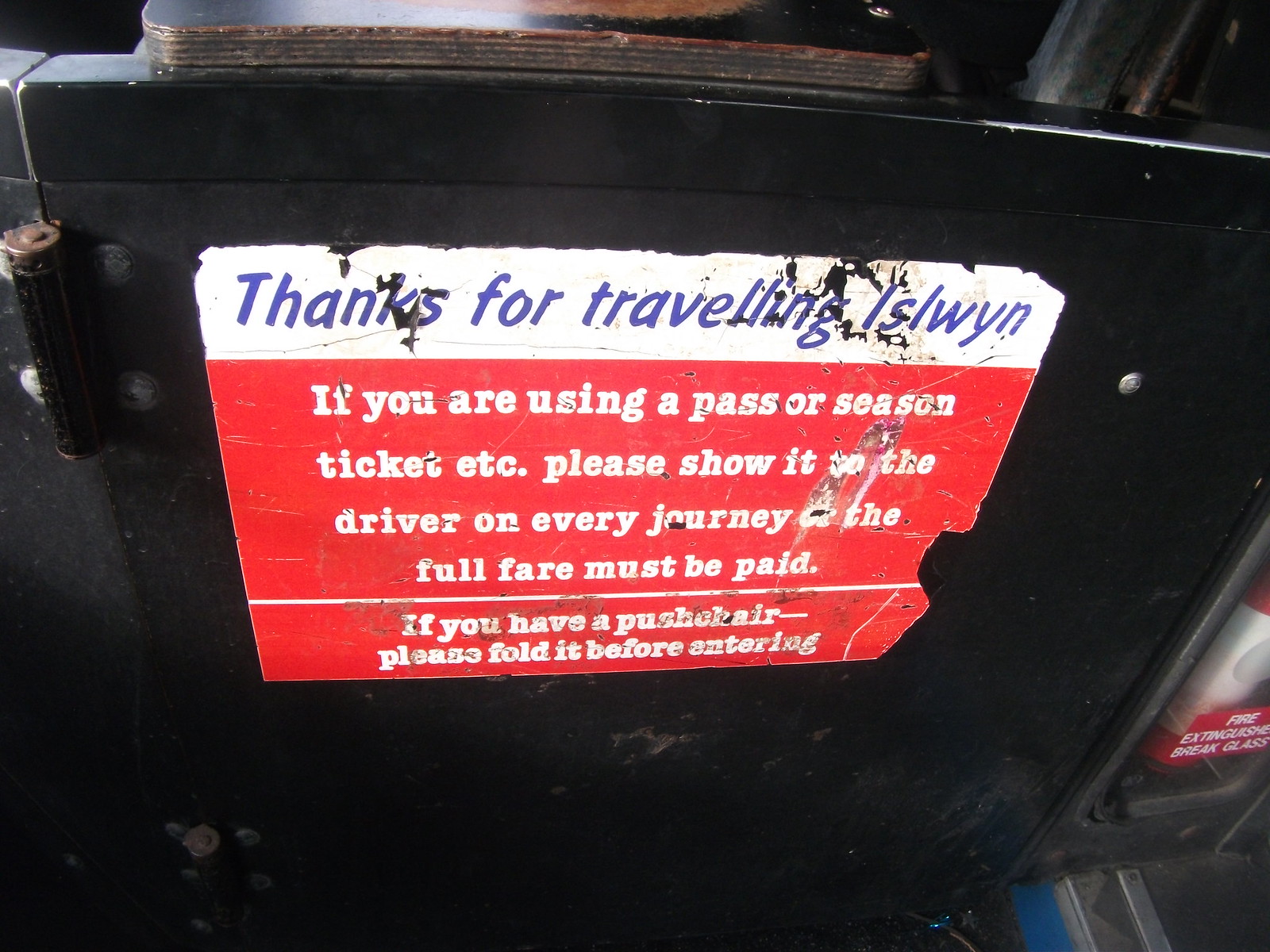The image features the back of a seat inside a worn-down tour bus or a similar public transport vehicle. The seat is made of dilapidated black wood that appears reinforced with screws to maintain its structure. Prominently displayed on the seat is an aged, frayed, and scratched sticker with noticeable chunks missing. The sticker contains instructions for passengers. At the top of the sticker is a white box with blue text that reads, "Thanks for traveling to Isilwin." Below it, housed within a red box with white text, the message advises, "If you are using a pass or season ticket, etc., please show it to the driver on every journey. The full fare must be paid." Further down, separated by a white line, it reads, "If you have a pushchair, please fold it before entering." Partial views of a fire extinguisher encased in glass and what looks like steps leading into the vehicle are visible to the side, suggesting the image is set near the entrance of the bus.